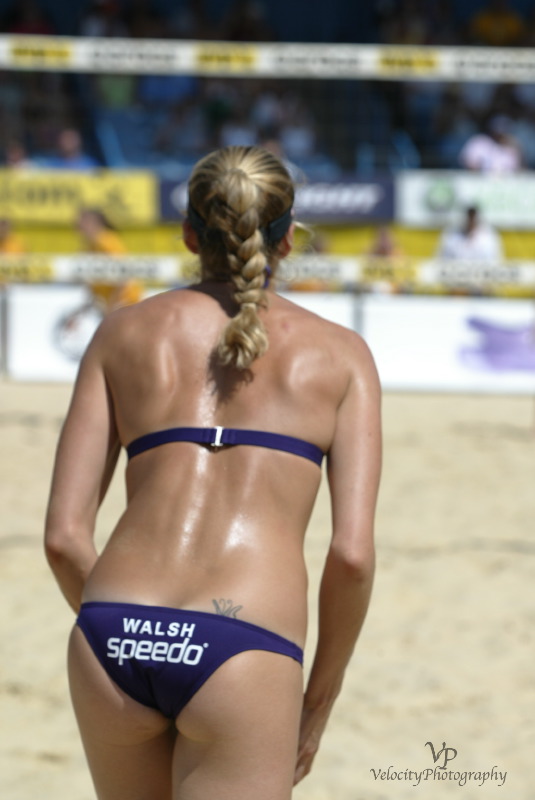In this photograph, we see an athletic woman on a beach, likely a professional volleyball player, captured by Velocity Photography (indicated by the watermark in the lower right corner). She stands with her back to the camera, showcasing her toned physique. Her hair is styled in blonde braids or a ponytail, and the sun shines down on her, illuminating her athletic build.

She is dressed in a minimalistic bikini; the top is strapless with a blue strap featuring a gold center, and the bottom is a purple pair of Speedo swimming trunks emblazoned with "Walsh Speedo" in white lettering. Above her right lower back cheek, she has a visible tattoo.

The scene unfolds on a sandy beach where she appears ready to play volleyball. In the background, a hazy, blurry volleyball net is positioned roughly 15 feet in front of her. Distant spectators are visible, seated behind a white barrier, adding to the beach event atmosphere.